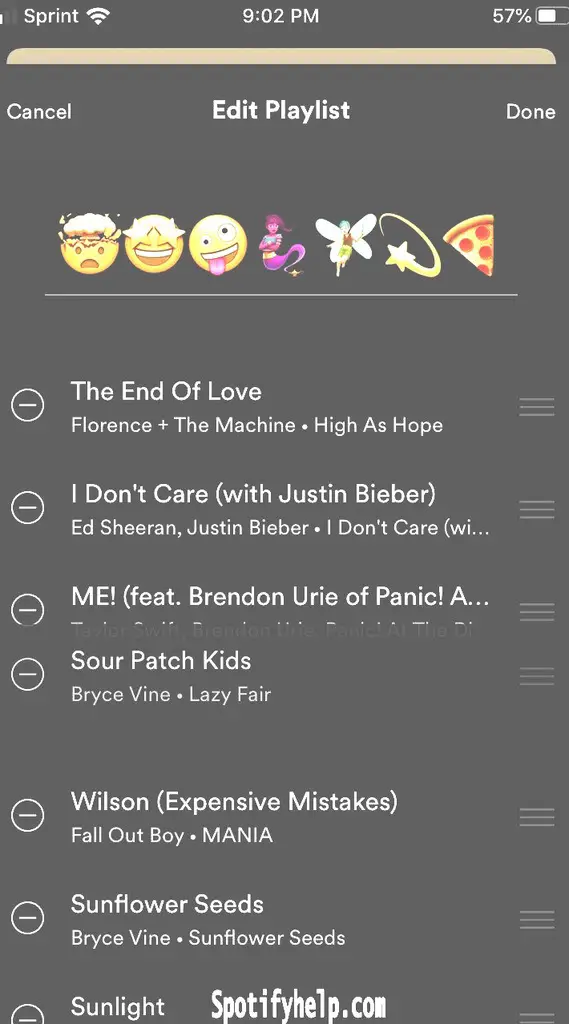The image displays a smartphone screen at 9:02 PM, showing a Sprint network with full WiFi signal and 57% battery life. The screen captures various playful and eclectic elements, including:

1. A header with an explosive head emoji followed by bright stars, a silly mouth emoji, a genie, a fairy, and a star.
2. A scattered array of pizza slices topped with pepperoni.
3. An icon depicting a circle with a minus sign, indicating "the end of love."
4. Mention of musical references such as "Florence + the Machine" and various song titles, including "Hi Asshole" and "I Don't Care" by Justin Bieber and Ed Sheeran.
5. Pop culture references including "Brendon Uriel" of Panic! at the Disco and Sad Patch Kids.
6. Text including "Brights Fine," "Lazy Faire," and "Wilson, Expensive Mistakes" by Fall Out Boy.
7. Mentions of snacks like "Sunflower Seeds."
8. The phrase "Spotify Hub.com."
9. A grey overlay on a Windows platform display. 

Captured on the phone screen are various elements indicating music playback, playlist editing, and expressive emoji-icons reflecting a mix of whimsical and humorous content.